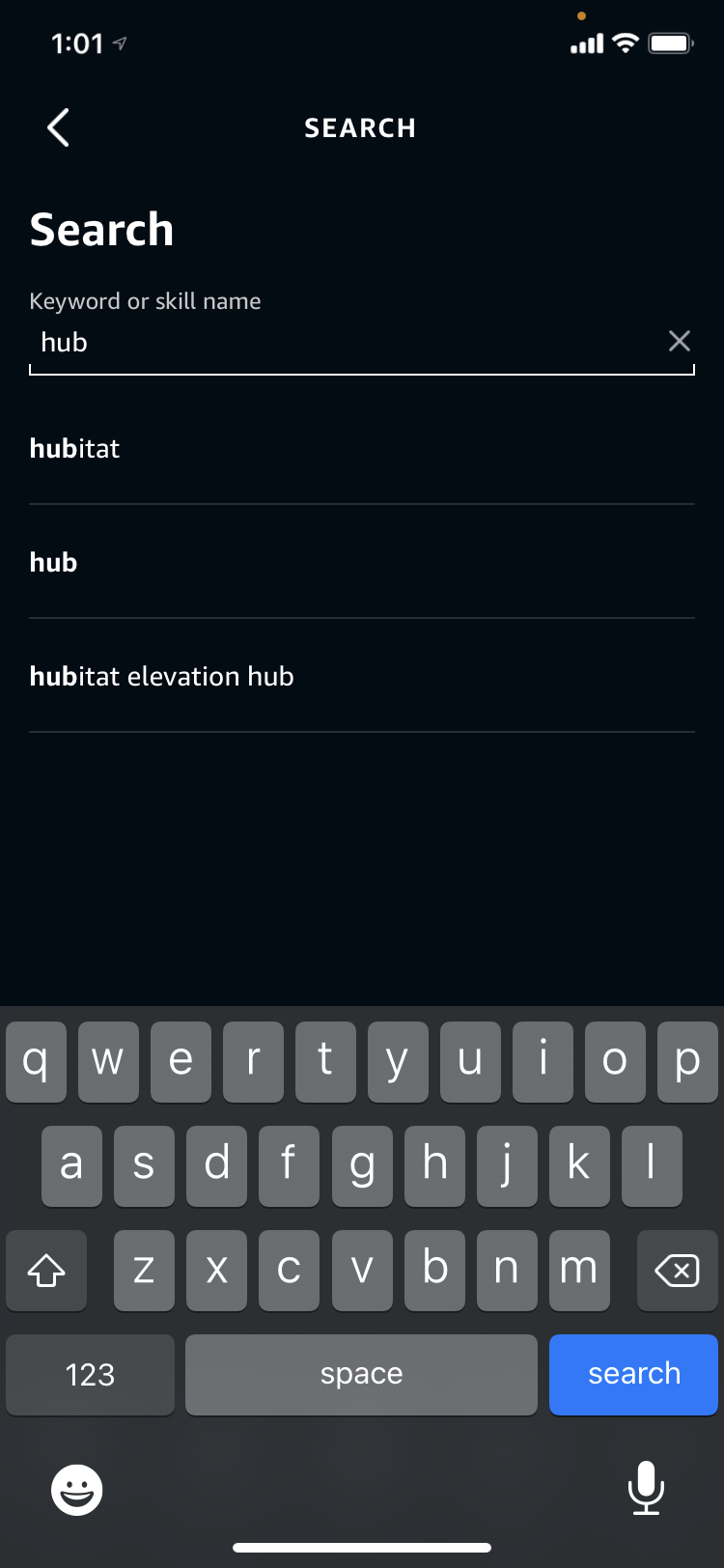This image is a cropped screenshot taken from an iPhone, depicting an app interface with a search feature. The background of the interface is predominantly black. At the top-left corner of the screen, the time is displayed as 1:01, accompanied by icons for signal strength, Wi-Fi connectivity, and battery level on the right-hand side.

Centered at the top, there is small text that reads "Search," followed by a larger text below it also stating "Search." Underneath, there's a text input box labeled "Keyword or skill name," and then a button labeled "Hub."

Beneath the input section, there are three search results listed:
1. Habitat
2. Hub
3. Habitat Elevation Hub

The lower portion of the screen features the iPhone keyboard. On the bottom-left corner of the keyboard, there is a white emoji icon, while the bottom-right corner displays a white microphone icon.